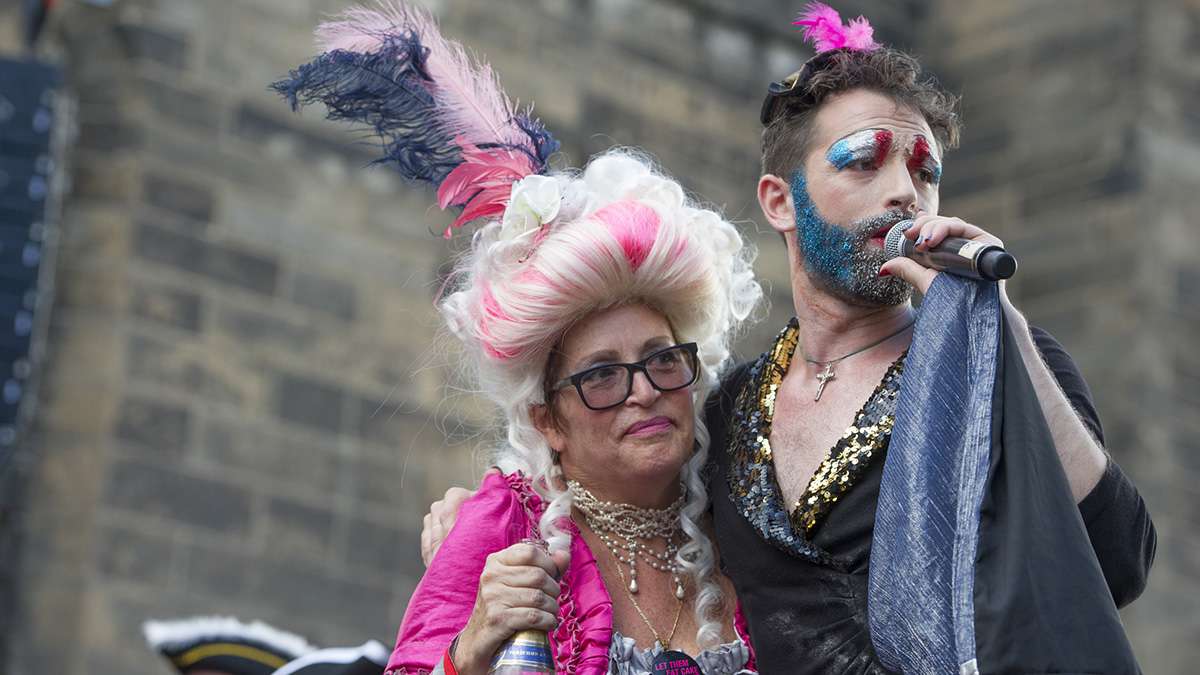In this close-up photograph, two individuals are dressed elaborately, exuding both a fancy and whimsical caricature-like charm which seems fitting for an exuberant event, possibly a gay and lesbian parade. The shorter person, presumably a woman, sports a voluminous colonial-style wig streaked with white and pink, accessorized with a large blue and pink feather. Her look is accentuated by black-rimmed glasses, pink lipstick, and a thick multi-layered pearl necklace that complements her Victorian-inspired pink jacket. Notably, she holds a bottle and wears a slightly frowning expression. Beside her stands a man, probably in his late 20s, with his arm around her. He has brown spiked hair adorned with pink feathers, and his beard painted blue and gold, matching his bold eyeshadow in red, white, and blue patterns. His ensemble includes a low-cut, tight black jacket embellished with gold and silver glitter, revealing a cross necklace. Holding a microphone, he appears to be speaking, adding to the lively and dynamic feel captured in the image. Both individuals stand against a masonry wall, looking off to the side, embodying a festive and vividly detailed scene.